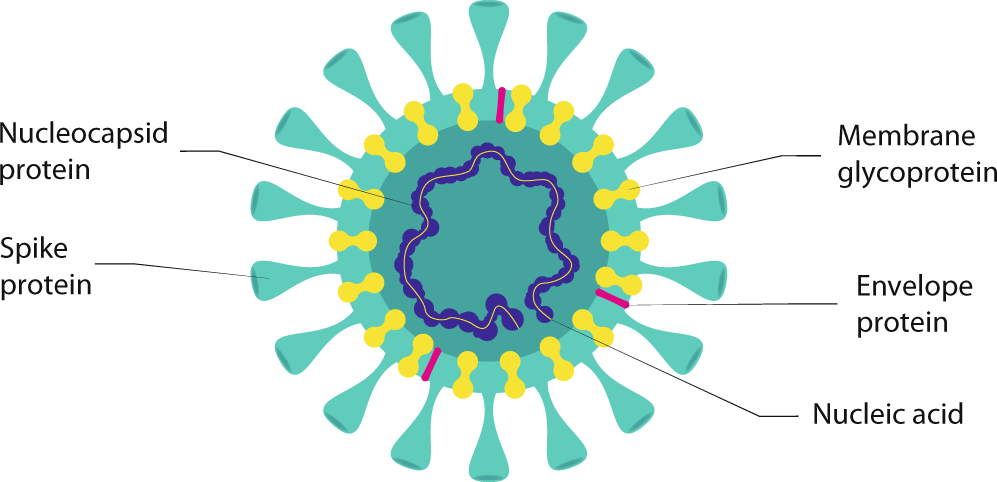This highly detailed medical diagram illustrates the structure of a microscopic viral body, likely a virus, presenting various proteins and nucleic acid components. The central focus is a dark green sphere with a lighter green border, surrounded by multiple green protrusions resembling upside-down Erlenmeyer flasks, arranged in a circular pattern, approximately twenty in total. The centrally located text labels include "Nucleocapsid Protein" connected via a black line to a dark blue, squiggly line in the core. "Spike Protein" points to one of the green flask-like protrusions on the sphere's exterior.

On the diagram's periphery, "Membrane Glycoprotein" is linked to yellow dumbbell-shaped structures embedded in the border, encircling the sphere. "Envelope Protein" labels the teal band around the sphere, and "Nucleic Acid" points to the core, identifying the orange line within the blue squiggle. Various colors highlight these components: green for the main body and spikes, yellow for the membrane glycoproteins, and blue and orange for the nucleic structures, emphasizing the complex molecular composition of the viral entity.